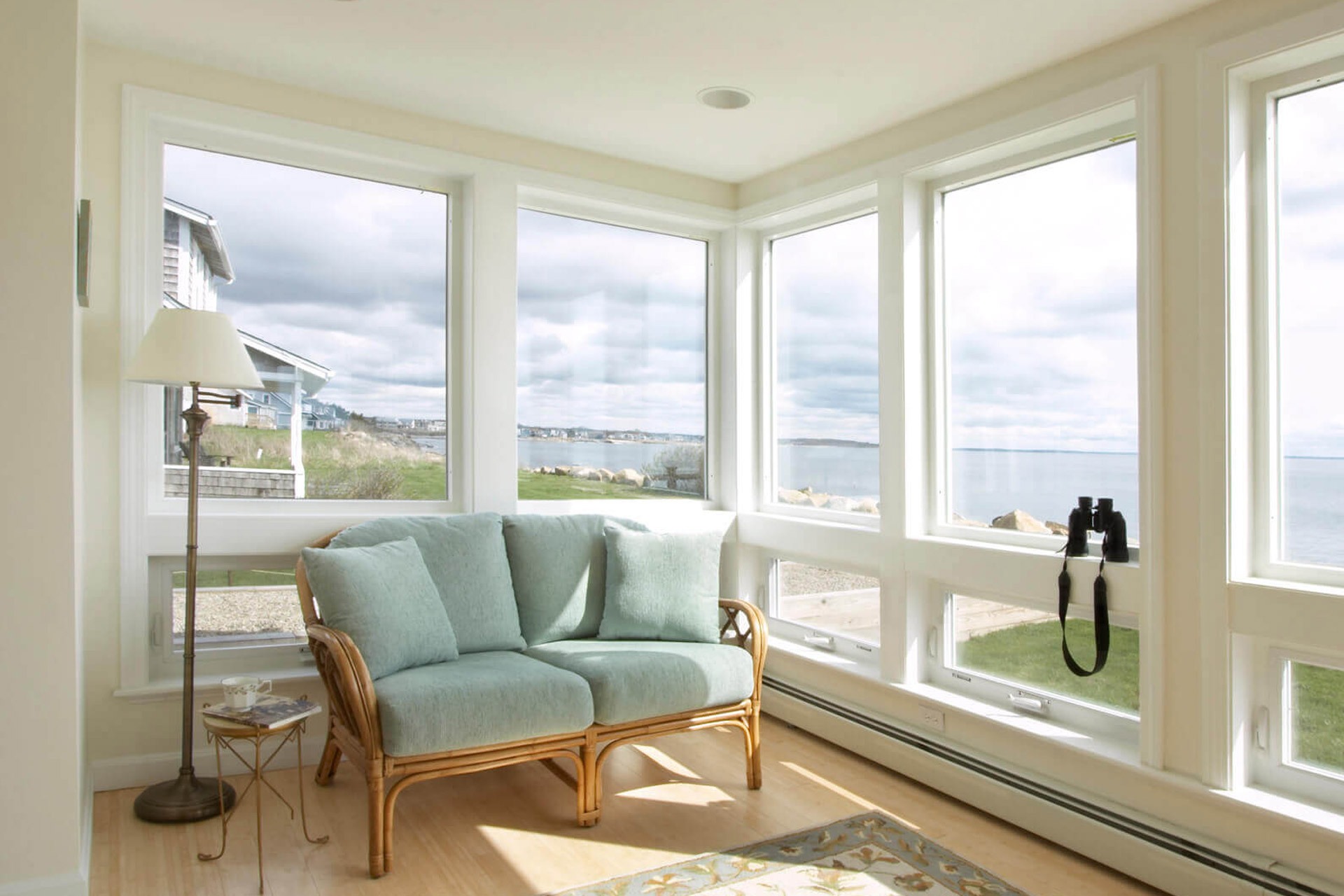This is a detailed interior shot of what appears to be a lake house, with a cozy corner prominently featuring large windows that offer a stunning view of a serene lake. The left wall houses a wooden bench designed to seat two people, outfitted with light seafoam green cushions along with matching pillows—a combination of backrest pillows and decorative ones arranged diagonally on the bench. Positioned beside the bench is a tall, thin, brown floor lamp with a white lampshade, casting a gentle glow over the area. A small side table matching the wooden bench stands nearby, holding a few books and a mug. On the windowsill, binoculars are carefully placed, presumably for viewing the picturesque outdoor scenery. Adding to the room's charm, a light green and brown rug is seen in front of the bench, complementing the calming, nature-inspired color palette of the space. The room itself is painted white, creating a bright and airy atmosphere that enhances the natural light flooding in from the ample windows. The inviting ambiance is completed with views of neighboring houses, grass, sand, and the water beyond, suggesting a tranquil lakeside retreat.